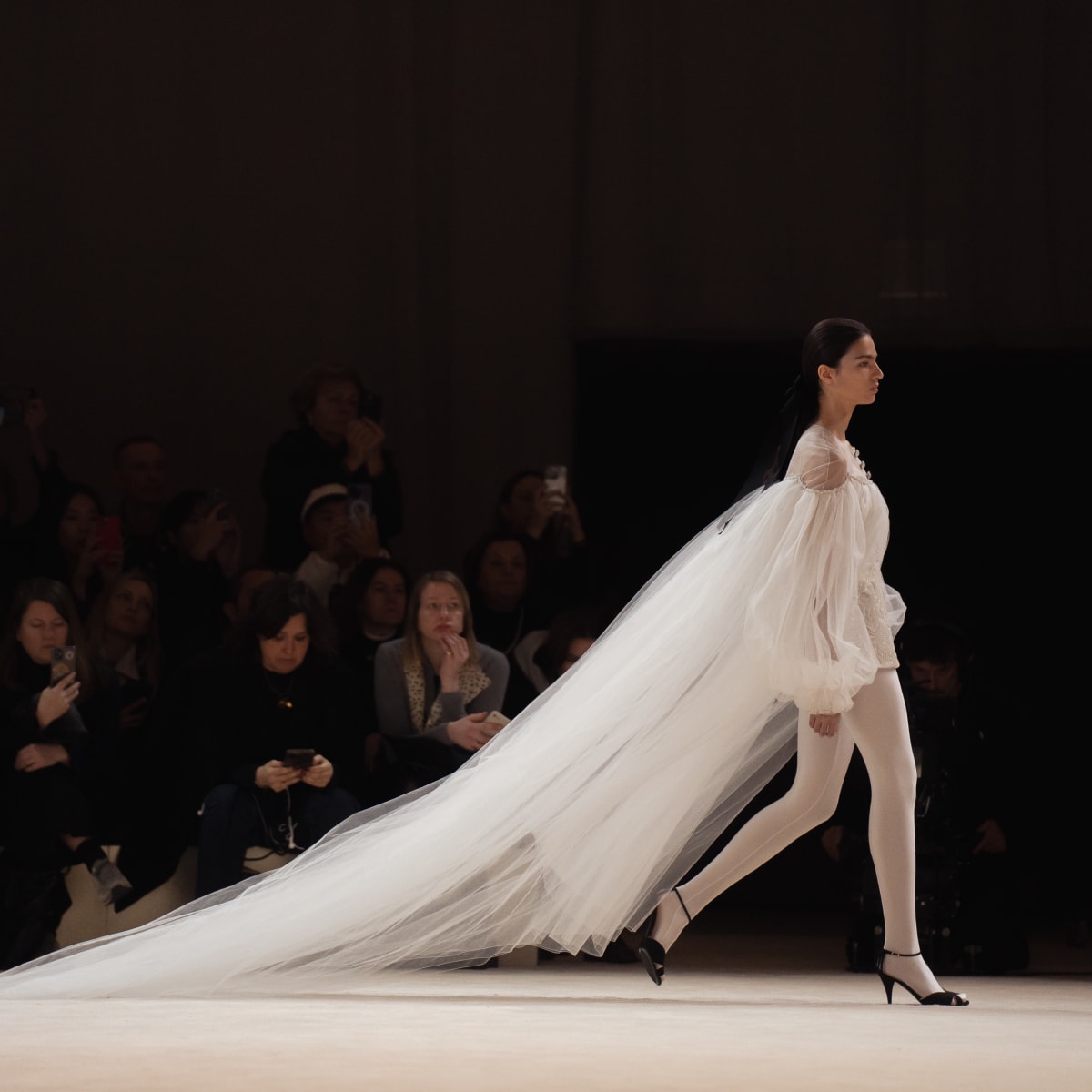In this striking image, we see a model striding confidently to the right on a pristine white runway. Her long, dark hair is pulled back, and she exudes poise with her neutral expression. She is adorned in an all-white ensemble, save for her striking black high heels, which feature pointed heels, ankle straps, and a slight open toe design. The outfit consists of a mini skirt paired with white stockings and a white lace top that reveals her shoulders. Flowing dramatically behind her is a long, voluminous veil or train, resembling bridal tulle, extending several feet from her shoulders and trailing elegantly along the floor.

The background features a white setting with walls, and the scene is further animated by the audience. Several audience members are captivated by the spectacle, some capturing the moment on their phones, while others watch in awe, with one person pressing her hands to her lips in fascination. The upper part of the background fades into blackness, highlighting the model as the focal point of this mesmerizing fashion display.